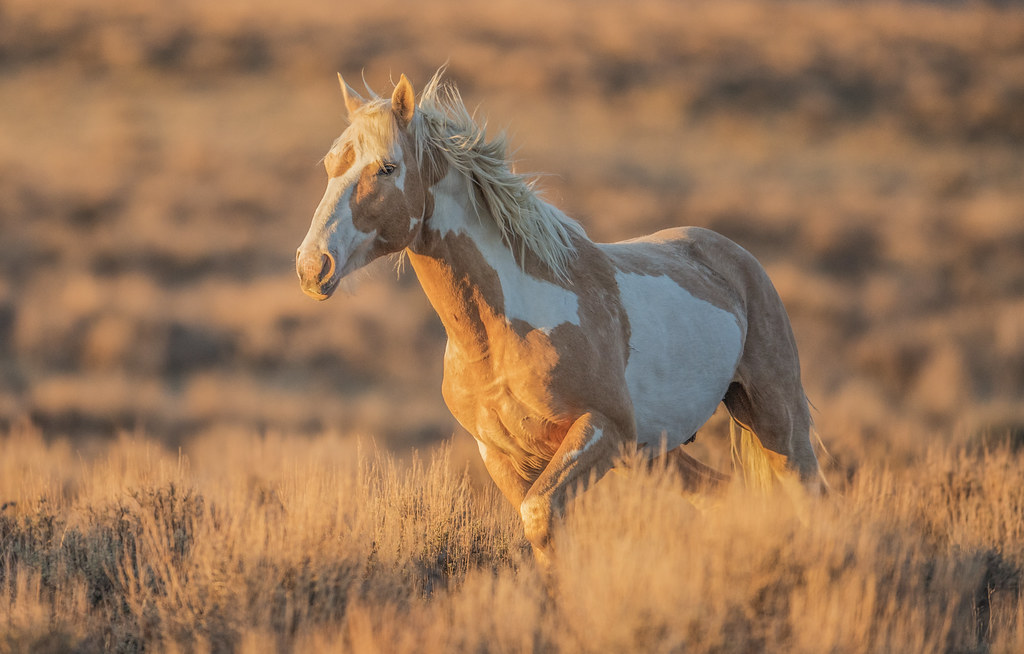The image captures a realistic photograph of a beautiful horse running through a field of high, dry, beige grass or hay. The horse, positioned centrally in the frame and running towards the left, features a striking tan and white spotted coat, with its blonde mane flowing messily in the wind. The horse's head is turned slightly to the left, with ears perked up straight, highlighting its alert and dynamic posture. You can discern its facial features distinctly, with white markings around its nose and eyes, complementing the prominent white patch on its neck and solid white undercarriage. The sun, low in the sky indicating either sunrise or sunset, casts long shadows and creates a vivid contrast of dark and light across the field. The background is artistically blurred but mirrors the beige tones of the foreground, with possibly more land or a hill subtly visible, adding depth to the serene landscape.